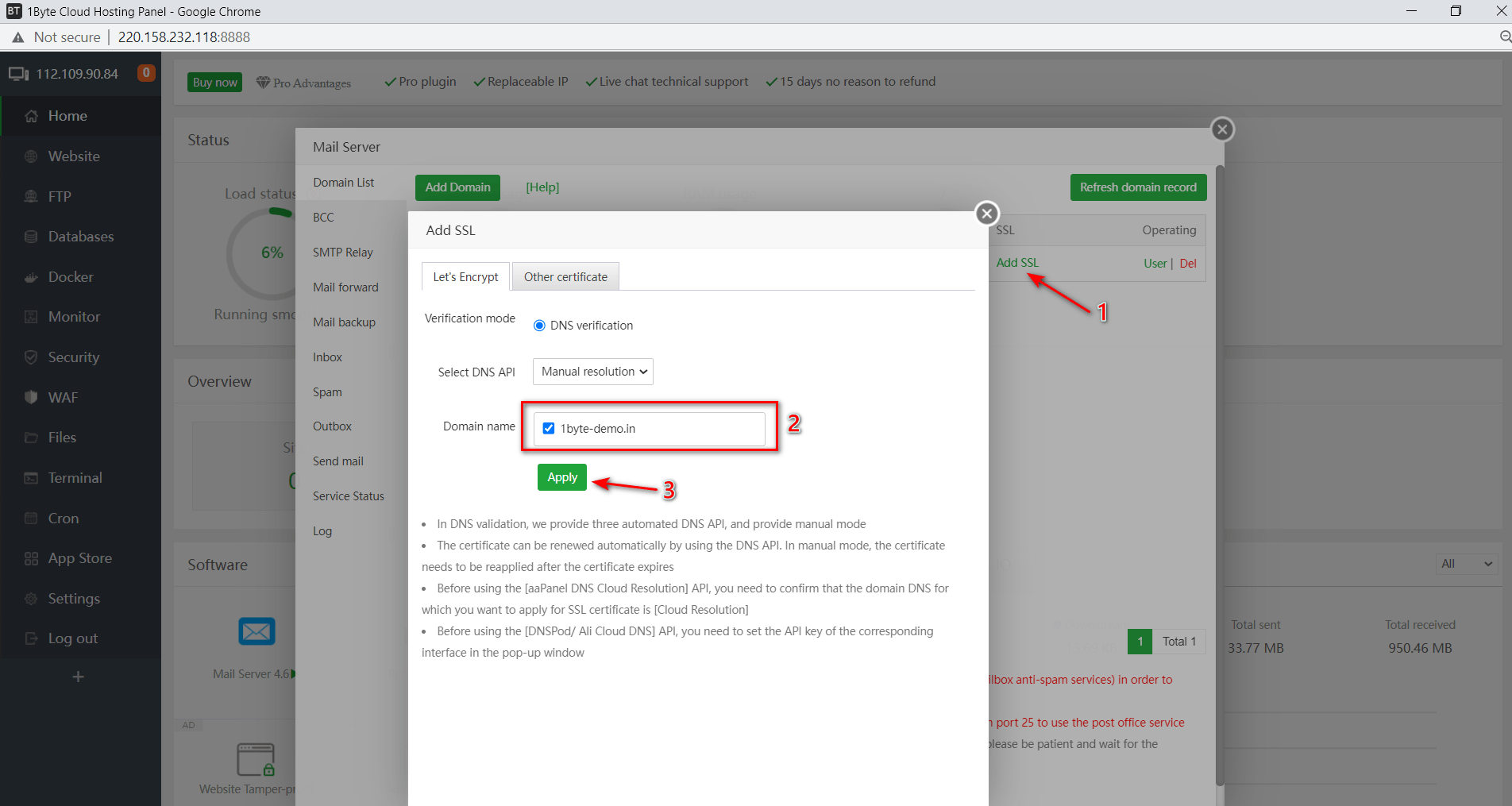A screenshot displays a web interface with a small, indistinct logo in the upper left corner that likely reads "BT" or "ET." The browser tab is labeled "1-byte cloud hosting panel - Google Chrome." Directly below, a warning triangle indicates "Not Secure," followed by the IP address "220.158.232.118:8888."

A vertical gray menu bar on the left lists the following options, each with an accompanying icon: 
- Home
- Website
- FTP
- Databases
- Docker Monitor
- Security
- WAF
- Files
- Terminal
- Chrome
- App Store
- Settings
- Logout

The main section of the screenshot is overlaid with two stacked pop-ups on a dimmed background. The smaller pop-up, partially visible, includes the following tabs: Mail Server, Domain List, BCC (Blind Carbon Copy), and various forwarding and backup options.

The larger, more prominent pop-up is labeled "Add SSL," offering options to "Let's Encrypt" or use "Other Certificate." It includes sections titled "Certificate Mode" and various unreadable texts. Beside the "Domain Name" field, there is a label marked "2" in a red rectangle. Below that, an "Apply" button is marked with a "3" and a green arrow pointing to it.